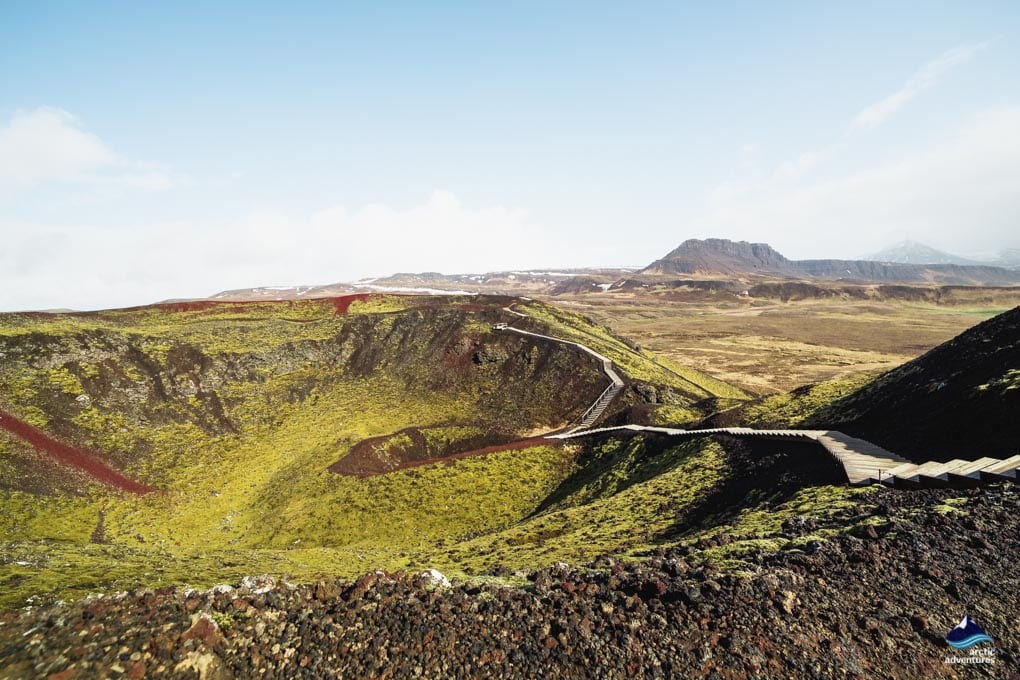This horizontal rectangular photograph captures a striking and desolate outdoor landscape dominated by a large crater, possibly a meteor impact site, situated on the center left. The crater features a bottom covered in light green vegetation and steep, rocky sides. A distinct white pathway, possibly a concrete stairway, descends into the depths of the crater, which suggests it may be accessible to tourists. Surrounding the crater are areas of dark soil and reddish terrain. On the left side of the image, the path leads downward near a mountain peak. The background reveals a vast expanse of flat land leading into distant, blurred mountains. Above this rugged scenery, a blue sky dotted with feathery white clouds stretches across the top of the photo. In the lower right-hand corner, there is a small image of a blue dolphin and the text "Arctic Adventures" in white print.